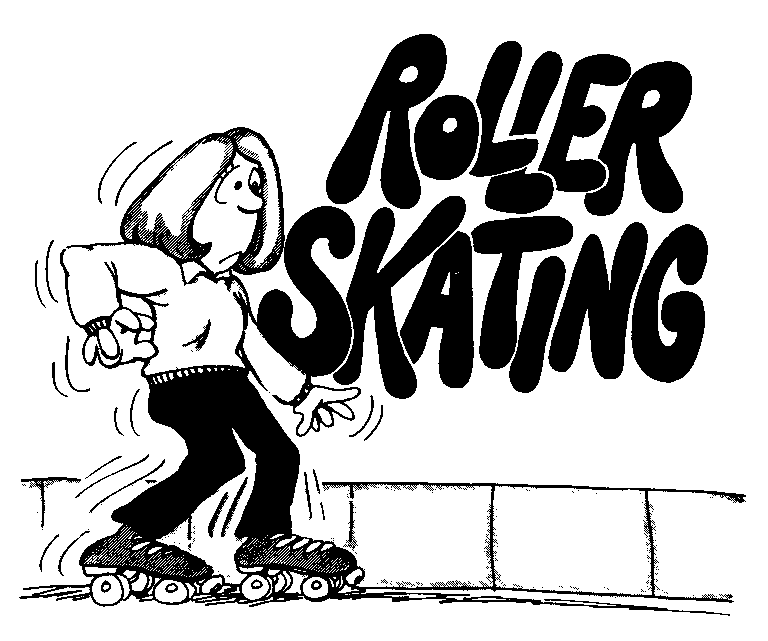The image is a black-and-white cartoon drawing without any visible borders, set against a plain white background and measuring approximately five inches tall and six inches wide. On the left-hand side, facing the right, is a cartoon depiction of a middle-aged woman wearing roller skates. She has shoulder-length bobbed hair, a frown, very wide eyes with small black dots as pupils, and pronounced eyelashes above her eyes. Her nose is pointy, enhancing her worried expression. She's dressed in a long-sleeve sweater with a collar; the sweater is depicted as white while her pants are black. On her feet are gray, four-wheeled roller skates.

The woman appears unsteady, as indicated by the shaky, curvy lines drawn around her arms and head to show movement. Her body language and facial expression suggest she’s anxious about losing her balance. At the bottom of the image, there is a small border wall, implying the scene takes place on a skating rink.

Dominating the right upper corner of the illustration, bold black bubble letters spell out "ROLLER SKATING," emphasizing the activity she's engaged in. The letters are all capitalized and add to the overall playful and exaggerated nature of the cartoon.